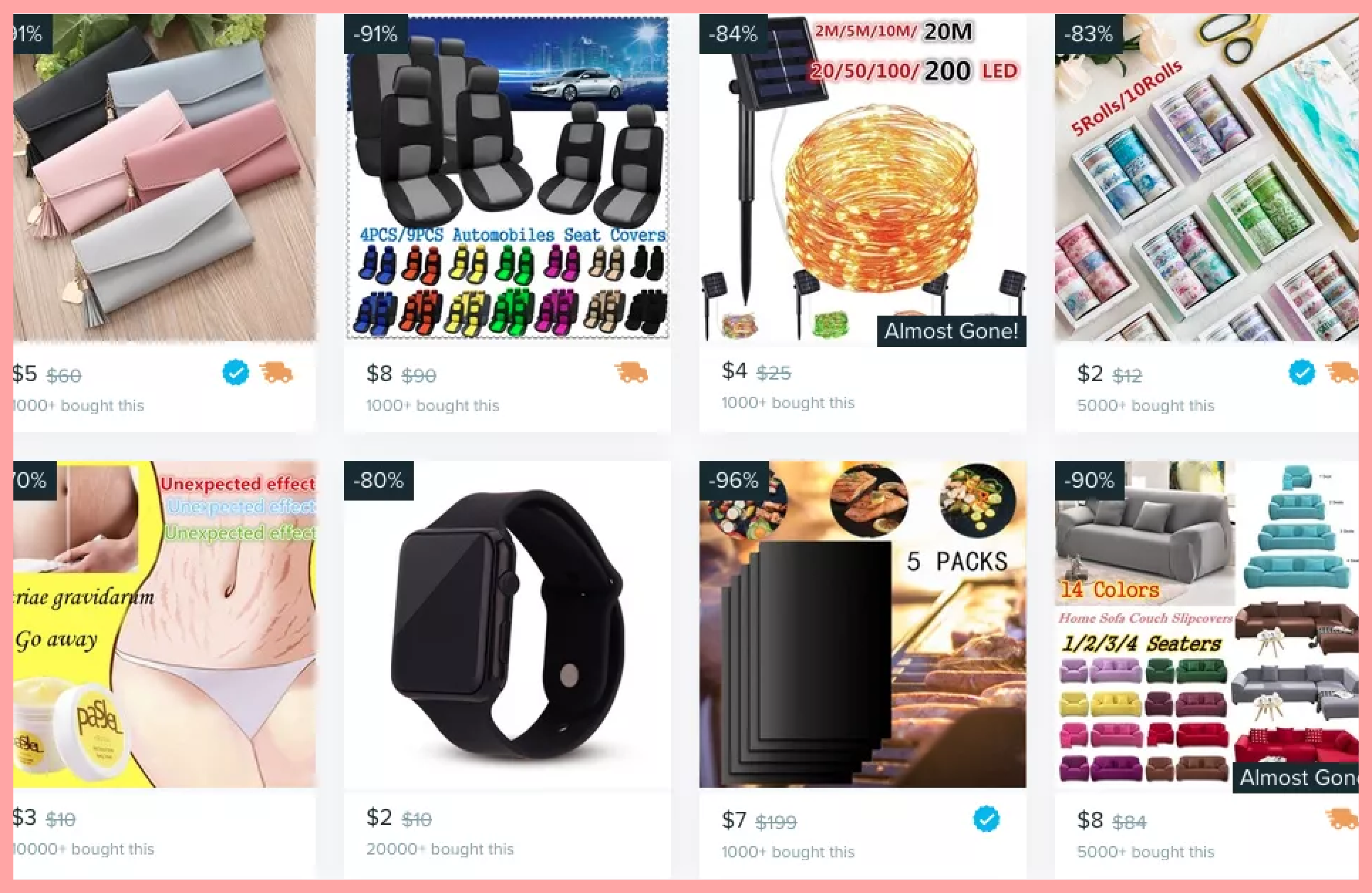A webpage displays an array of eight products arranged in two rows of four, predominantly characterized by their low prices and potentially questionable quality, reminiscent of platforms like Timu or Wish. At the top left, a collection of wallets is prominently featured, each priced at $5. Adjacent to them are car seat covers available for $8. The third item on the top row is decorative gold wire lights offered for $4, ideal for creating a twinkling ambiance. Completing the top row, a somewhat ambiguous product labeled as rolls, possibly small contact paper, is advertised in quantities of 5 and 10.

On the bottom row, the first item appears to be a cream aimed at reducing stretch marks, priced curiously at $3. Next in line is a watch that resembles an Apple Watch but is priced at a mere $2, clearly indicating it’s a replica. Following this is an unclear item presented as "5 packs" with illustrative food images above; only the price of $7 is certain. Lastly, the row concludes with a visually colorful couch being offered at $8, an eyebrow-raising deal for furniture.